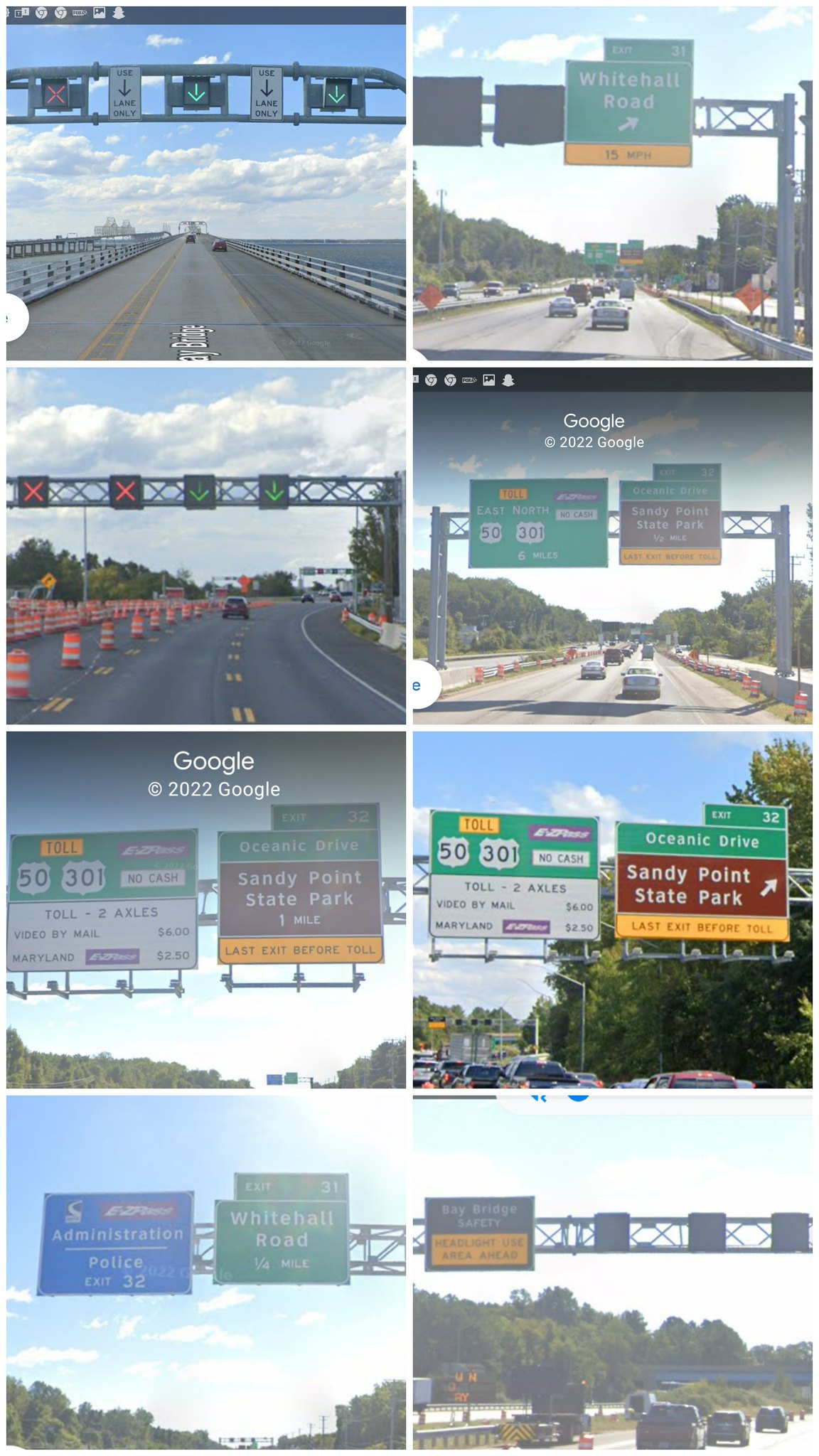This rectangular image, resembling the layout size of a cell phone screen, features a grid of eight small photographs arranged in two columns and four rows, each depicting various roads and highways.

In the upper left corner, there's an image of a bridge spanning over a body of water during daytime. Adjacent to it, on the right, is a photograph of a two-lane highway with a sign that reads, "Exit 31, White Hall Road."

In the second row, the left image showcases a three-lane highway, while to its right, there's a picture labeled "Google 2022" that indicates "Exit 32, Sandy Point State Park."

The third row, on the left, contains another "Google 2022" labeled image which details toll information: "EZ Pass, no cash for Roads 50 and 301," with a fee of "$6 for a two-axle, $2.50 for a Maryland EZ Pass." To the right, there's another photograph of Sandy Point State Park.

In the bottom row, the left-hand side image displays a sign that reads "EZ Pass Administration." Next to it, on the right, is an image of White Hall Road. Finally, in the lower right corner, there's a picture of a freeway or parkway with cars traveling in both directions and a sign that instructs, "Bay Bridge Safety, Headlight Use Ahead."